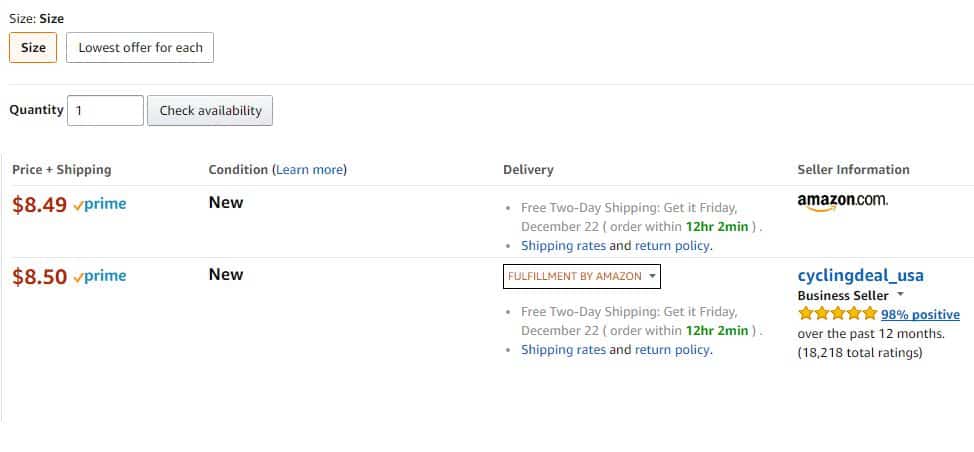In this screenshot of an Amazon page, the right side of the upper corner displays seller information. Below this, the Amazon.com logo is prominently displayed, followed by the seller name in blue text. The seller is a business entity based in the USA, offering a current selling deal. The seller has an impressive rating with five yellow stars, boasting 98% positive feedback over the past 12 months, accumulated from 18,218 total ratings. 

To the left, delivery details are highlighted, stating "Free two-day delivery", with an expected arrival date of Friday, December 22nd if ordered within 12 hours and 2 minutes. Information about shipping rates and the return policy is also provided. Below, an action pull-down box indicates that the order is fulfilled by Amazon. Further down, the details about the free two-day shipping reiterate, mentioning the same expected delivery date of Friday, December 22nd, contingent on ordering within the same timeframe, along with shipping rates and return policy. 

The layout succinctly organizes crucial purchasing information, making it easily accessible for potential buyers.